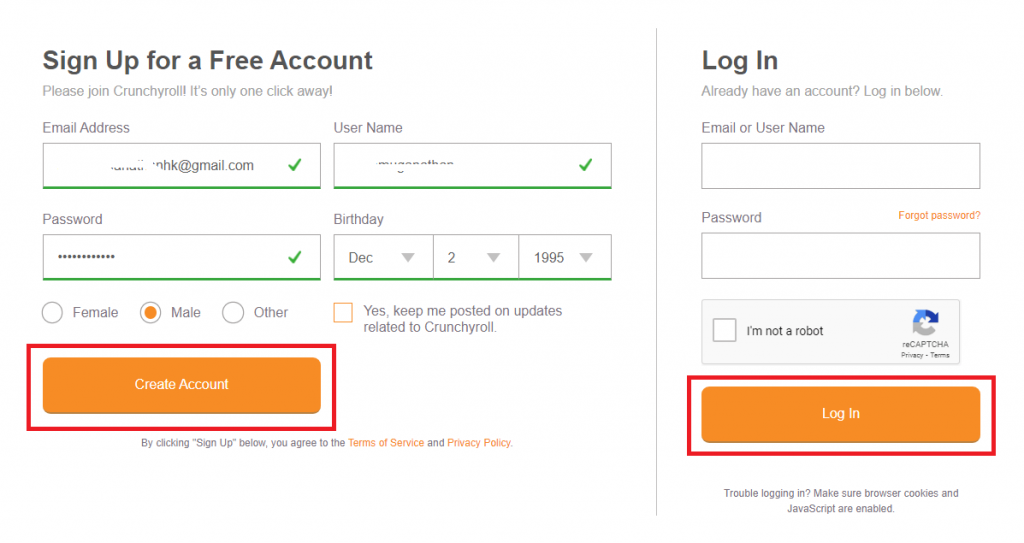The image depicts two screenshots side-by-side, centered and framed for clarity. Both screenshots are related to an account creation and login process on a website with a white background.

The left screenshot appears to be a sign-up form for creating a new account on Crunchyroll, a platform for streaming anime and other content. The form is titled "Create Your Free Account" and includes fields for username, email address, password, and birthdate, each underlined in green. The highlighted section in the center of the screen is encased in a red rectangle, emphasizing where users need to input their details. The form also features checkboxes for agreeing to terms, choosing whether to receive emails, and other options.

The right screenshot displays the login form for existing users. The title "Already Have an Account? Login Below" is prominently shown above the input fields. Users are required to enter their email or username and password, with a "Forgot Password?" link for those who need assistance. Below these fields, there is a "I'm not a robot" CAPTCHA and a "Login" button, the latter highlighted within a red rectangle, drawing attention to its importance.

Both forms are presented on a clean, white background to provide a seamless and user-friendly interface.